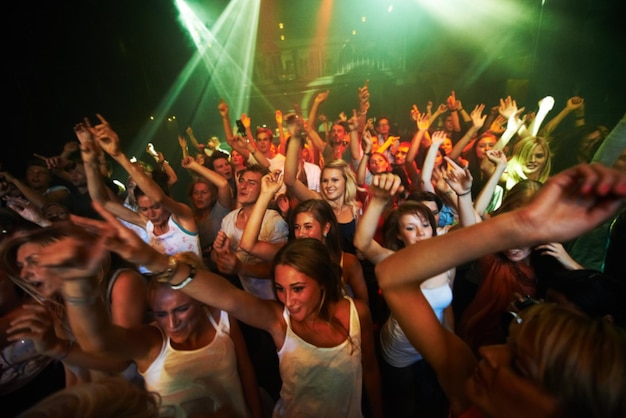The image captures the vibrant energy of a concert crowd from an overhead viewpoint, focusing on a sea of mostly young women, with a sprinkling of young men, all dressed in white tank tops and shirts. Their faces are lit up by a mix of green and red stage lights that pierce through the dim atmosphere, highlighting their animated expressions and movements. Most of the attendees, about 30 or so, are packed closely together, extending around eight or nine rows deep. The excitement is palpable as many of them have their arms raised, primarily their right hands, moving in rhythm with the music. Some are caught in moments of euphoria, mouths open in screams of joy, while others are smiling broadly and swaying. Despite not seeing the performer or stage directly, the photo perfectly captures the electrifying ambiance and communal thrill of the concert, underscored by the neon hues illuminating the enthusiastic crowd.